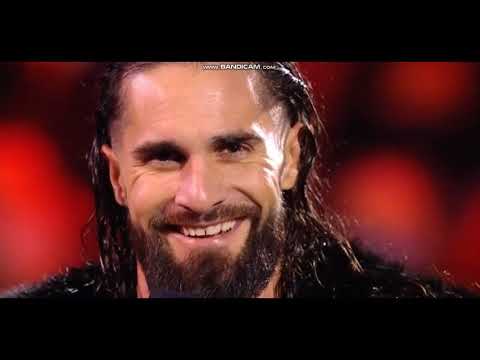A close-up photo captures a smiling white man with long, dark, and slightly greasy hair that is slicked back, revealing a mustache and a full beard. His dark brown eyes have smile-induced wrinkles, the left eye more illuminated due to the light source. He dons a black garment that looks fuzzy, possibly a fur jacket, visible only up to his shoulders. The man faces the camera directly, exuding a slightly mischievous expression. Behind him, the background is black with indistinct red circles or neon lights, suggesting an interview setting. Additionally, the image features black horizontal bars at the top and bottom, with white text at the top center reading "www.Bandicam.com," indicating the video source.